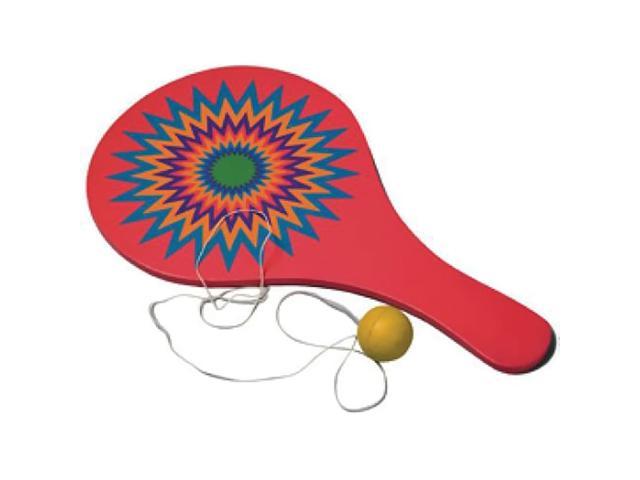This image features a vividly colored children's paddle ball toy primarily composed of a red paddle adorned with an intricate sunburst or explosion pattern. The paddle is positioned diagonally with the handle in the bottom right and the broader part in the top left. This colorful design is layered with various hues: an outer blue ring, followed by orange, purple, dark orange, blue again, and green, converging into a central green circle. A curly white string extends from the bottom of the paddle, attached to a yellow or light greenish-gold rubber ball with a ridge around its center. The background is plain and white, emphasizing the detailed, playful appearance of the vintage-inspired paddle ball toy.